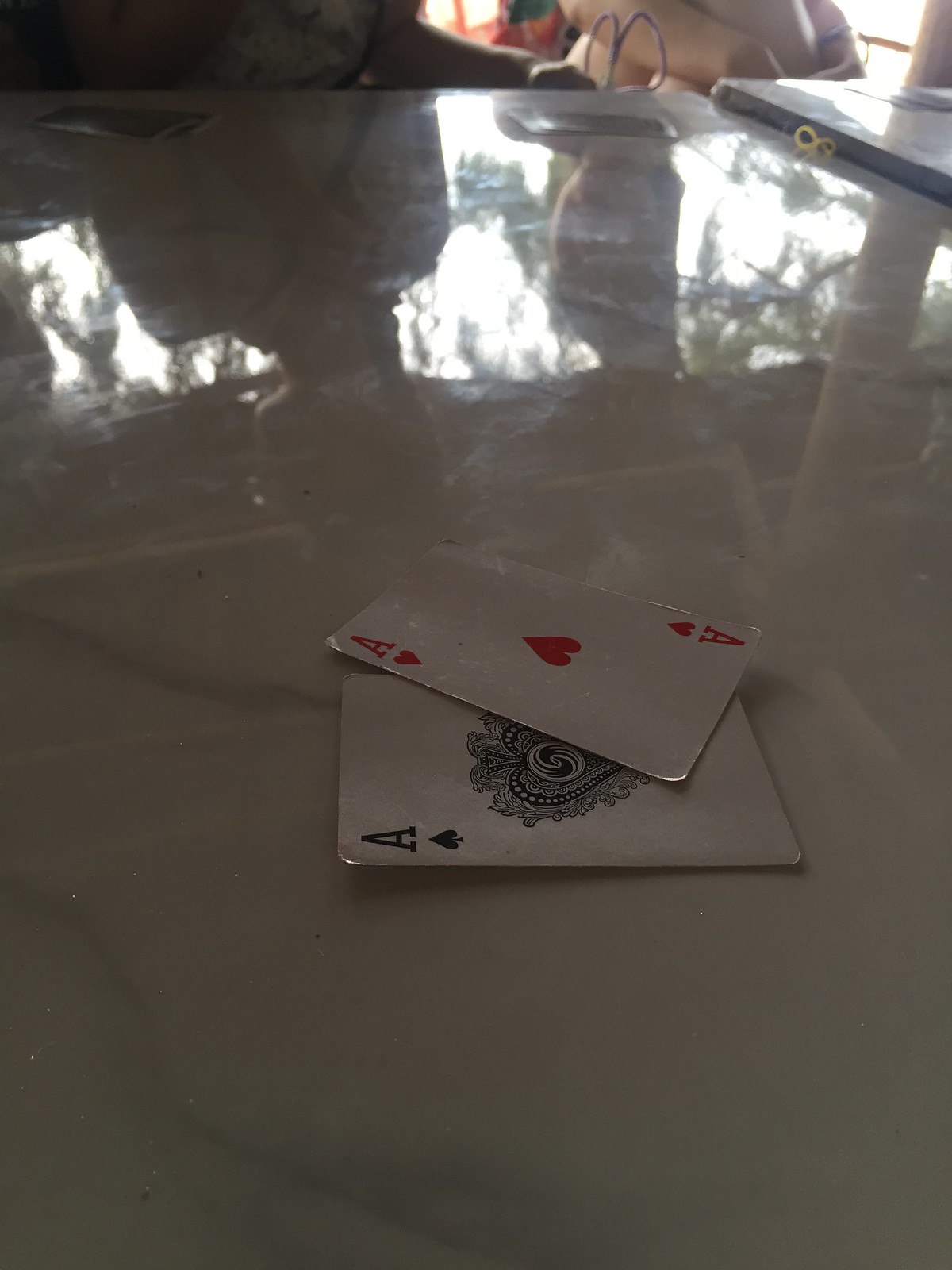In this photograph, we observe a dimly lit outdoor setting, discernible from the faint reflection of the overcast sky on a marble-top table that dominates the image. The table, exquisitely polished and pristine white with delicate gray marbling, gleams under the ambient light. A human reflection occupies the upper left corner of the table, hinting at a person seated nearby. While specific details about the individual, such as age or gender, remain indistinct, you can see a shadowy glimpse of their arm and torso. 

The focal point of the image is the two playing cards laid on the lower center of the table. An ace of spades lies flat with the 'A' facing to the left, showcasing a central spade design. Overlapping it slightly, the ace of hearts is similarly oriented but tilted a bit more towards the upper left corner. The overall composition, with its mysterious reflections and meticulously arranged cards, evokes a serene yet enigmatic ambiance.